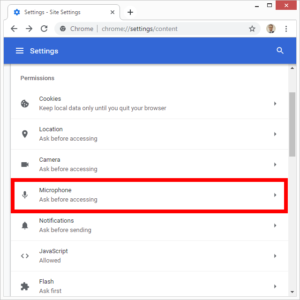The image captures a screenshot taken on a device while viewing the settings page of Google Chrome. At the top of the screen, "Settings" is prominently displayed inside a royal blue rectangle. This title bar features three horizontal bars (indicative of a menu) on the left and a magnifying glass (representing a search function) on the right, both icons in white. 

As the eye moves down the image, various permissions categories are listed, including Cookies, Location, Camera, Microphone, Notifications, JavaScript, and Flash. The "Microphone" section is highlighted with a red rectangle. Inside this red rectangle, the section shows a microphone icon next to the word "Microphone," followed by the phrase "Ask before accessing." To the far right of the "Microphone" section, there's a rightward-pointing arrow, indicating additional settings or details can be accessed. 

The middle portion of the screen is a blank white area, emphasizing the clean layout. On the far right side of the image, a scrollbar is visible, suggesting there are more settings that can be viewed by scrolling down.

The overall focus is drawn to the "Microphone" settings due to the red rectangle, emphasizing its importance or relevance in the context of the screenshot.